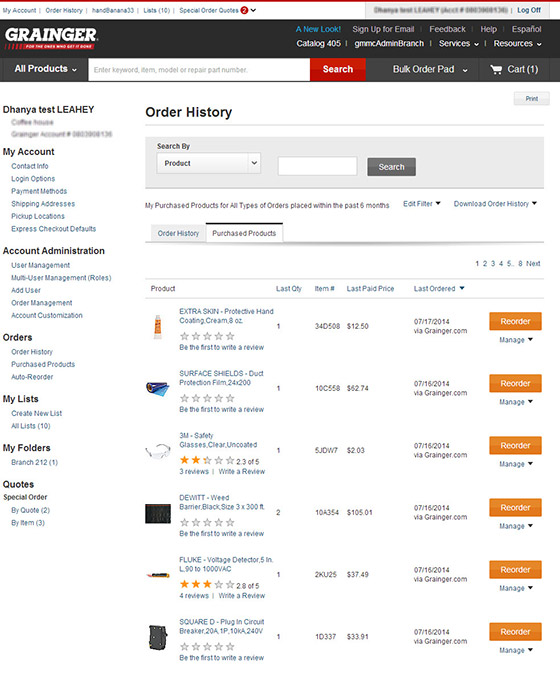The screenshot captures an e-commerce website selling a variety of products. At the very top of the page, black text reads "My Account," followed by "Order History." Further to the right, an indecipherable username is listed next to "Lists (10)," and then "Special Order Quotes." The top right corner features a gray button with blue text labeled "Log Off."

Directly beneath this is a very dark gray banner. On the top left of the banner, bold white block text spells out "Granger." Below this text is a narrow red stripe containing unreadable white text. In the top right of the dark gray banner, several options are listed: "Espanol," "Help," "Feedback," "Sign Up for Email," and a "New Look" notice, all aligned from right to left. Below these options, also from right to left, are "Resources," "Services," "GMMC Admin Branch," and "Catalog 405" written in white text.

The banner also features a drop-down menu labeled "All Products" and a user input field for searching the store. Next to these are a "Bulk Order Pad" drop-down menu and a shopping cart icon denoted as "Cart (1)."

The left sidebar lists various links from top to bottom, including "My Account," "Account Administration," "Orders," "My Lists," "My Folders," and "Quotes," each with their own subcategories.

The central section of the page showcases a list of products corresponding to the user's order history, which is highlighted at the top of the page.